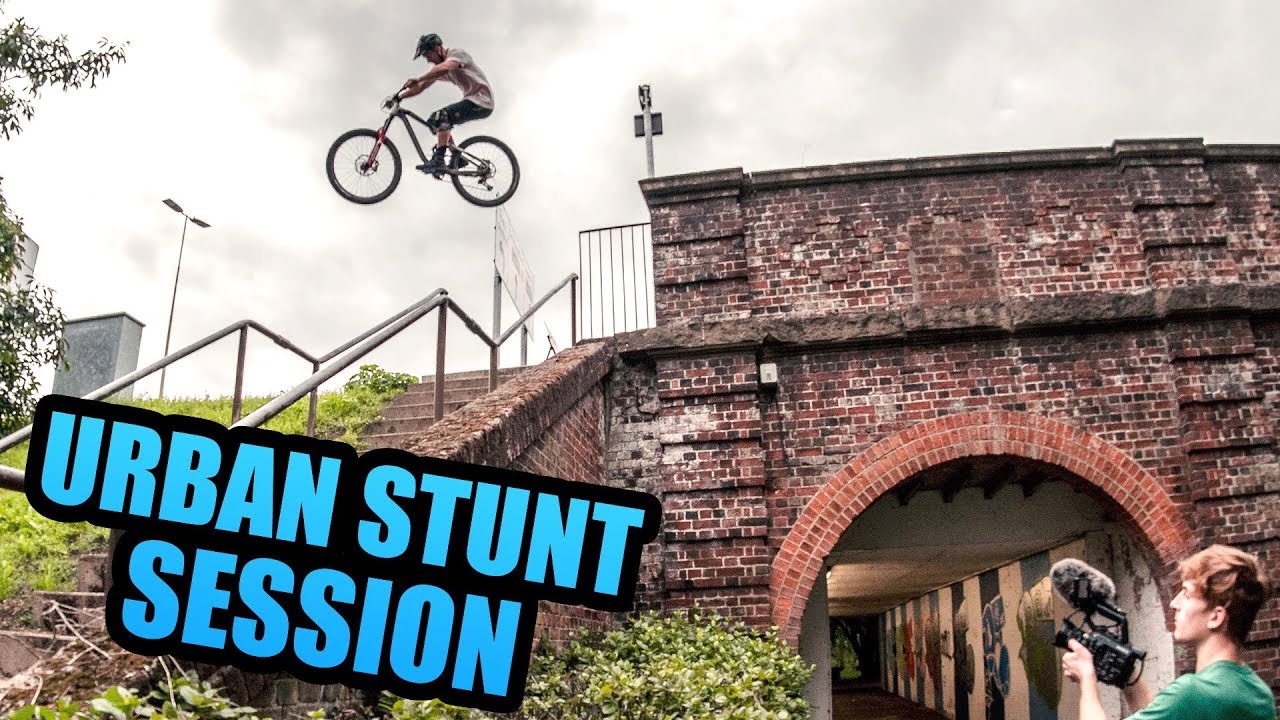In this vibrant and action-packed photograph, a young man wearing a helmet and knee pads is captured mid-air performing a daring bicycle stunt. He is seen jumping from a red-brick overpass, its aged structure featuring an archway and surrounded by greenery, including tree branches and bushes. The overpass, which functions as a bridge, has a staircase leading up to it, and a tunnel running underneath. In the background, you can spot a high-rise building and streetlights. On the ground in the right-hand corner, another individual is recording the stunt with a video camera. The image, framed in a wide rectangular format, showcases the words "Urban Stunt Session" in bold blue letters in the bottom left-hand corner, underlining the intense urban biking scene.